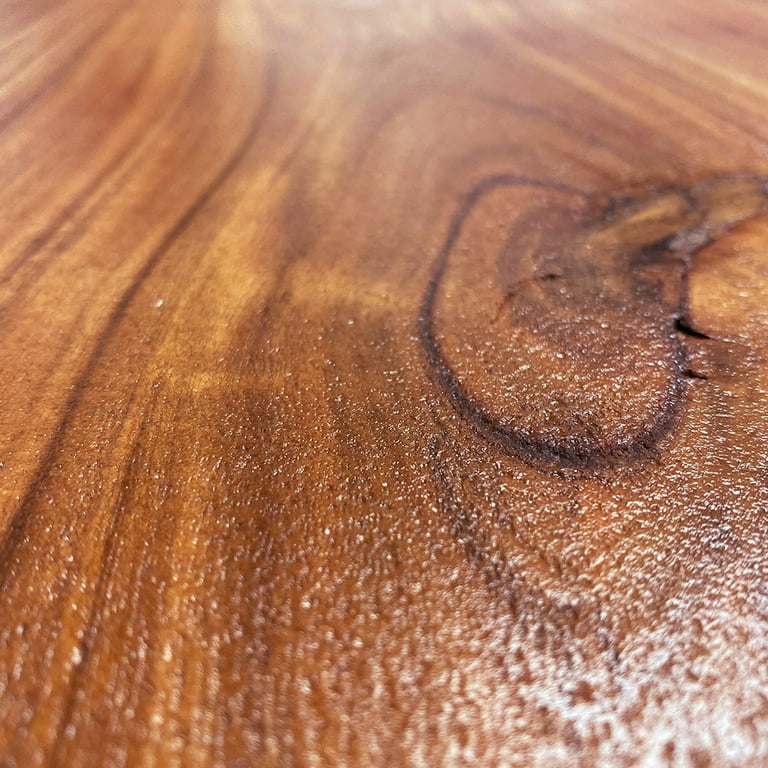This extreme close-up image showcases a piece of varnished wood, possibly from a tabletop or flooring. The wood, predominantly a gradient of light to dark brown hues, features intricate grain patterns. The left side of the image appears lighter, possibly due to reflected light. A prominent knot near the center-right stands out with its almost black ring, adding to the wood's natural character. The grain ascends and curves slightly, with some lines being notably darker, including one curving rightward from the bottom left. The bottom right highlights the wood's glossy, polished surface, reflecting light and revealing its textured, clean finish, dotted with tiny natural holes.